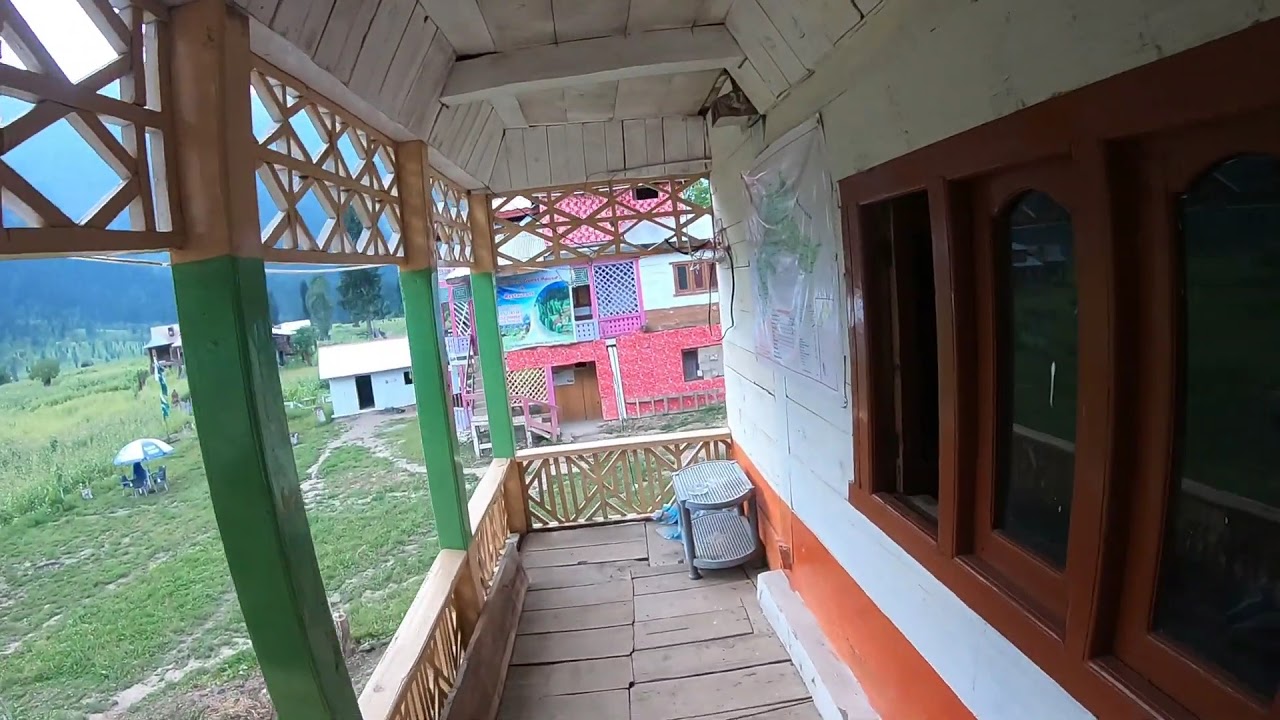This photograph depicts a detailed view of a balcony area of a house taken during daytime. The balcony itself is constructed of brown wooden slats that form the floor, giving it a rustic feel. The railing of the balcony is cream-colored, with green-painted columns providing support. On the balcony, there's a small plastic table adding a functional touch to the space. 

To the right, the house wall is white, featuring a brown window, with the lower portion of the wall painted red. There are three windows with wooden panes; the one furthest in front is open, allowing a glimpse inside. Above, the porch roof or ceiling is made from white wooden slats.

On the left side of the balcony, one can view the outside, revealing a grassy yard dotted with a couple of chairs and an umbrella, and extending further to other houses. The nearest neighboring house, painted in pink and white, lies beyond the end of the porch. Three rectangular columns support the overhang of the porch, with light brown wooden slat work at the top and bottom, enhancing the structural elegance. Overall, the image captures a cozy and inviting outdoor space, seamlessly blending various elements and colors.